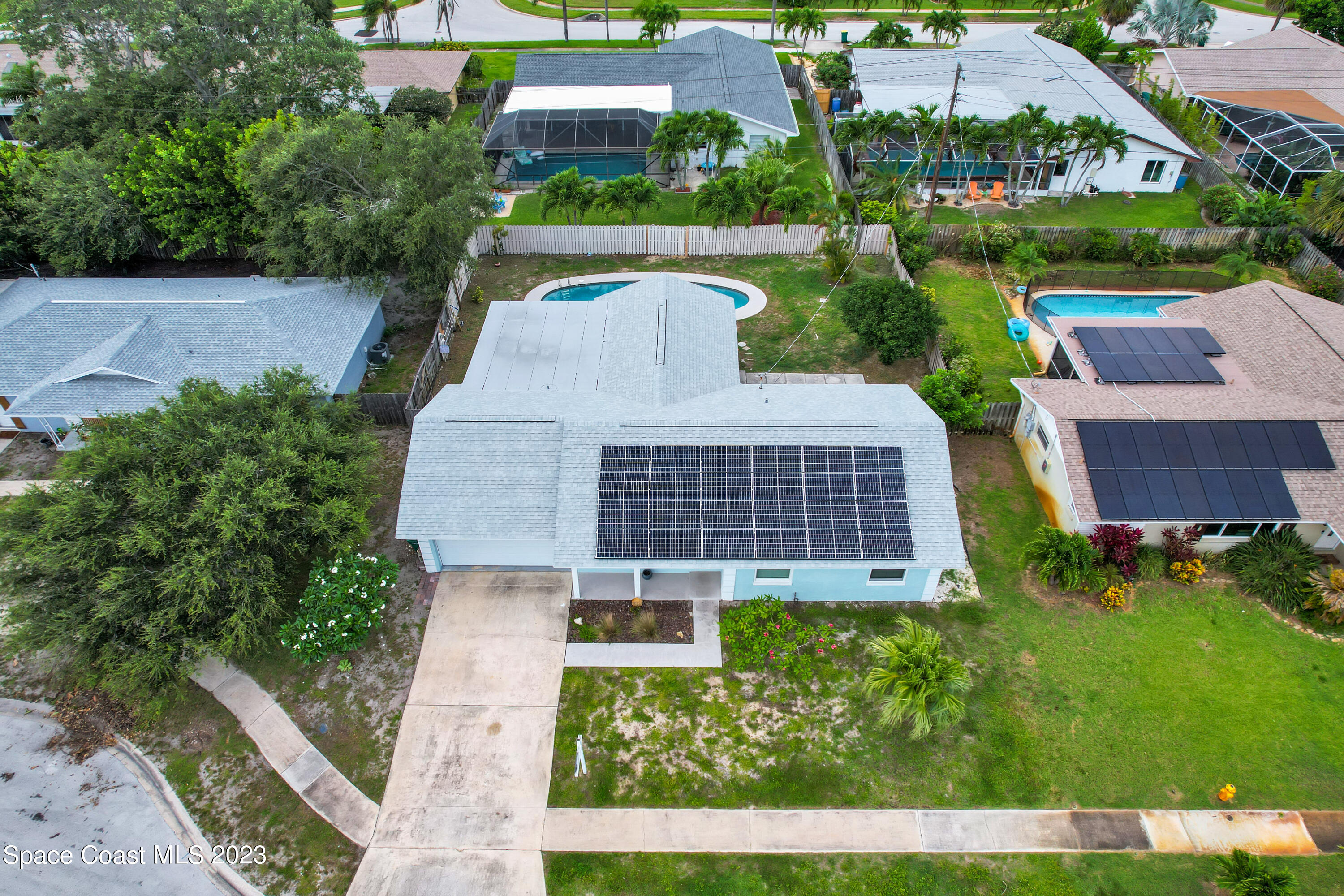The image presents a bird's eye view of a suburban housing estate comprising six visible houses, separated by patches of green grass, trees, and a network of pathways. In the top left corner, lush green bushes and trees frame a cobalt grey-blue roofed house. Below this house, a path can be seen stretching from the left side of the image, leading to a driveway in the bottom center, and heading back up towards another squarish house with a similar grey-blue roof. This house, located near the center, features black solar panels outlined in grey at its bottom and has a swimming pool at the rear.

Adjacent to this house on the right, there's a brown and beige roofed house, also equipped with solar panels and a swimming pool. Further up towards the top center of the image, another house with a light blue roof, lacking solar panels and a swimming pool, stands prominently. Left of this light blue-roofed house is yet another house with a dark blue-grey roof, furnished with solar panels and a swimming pool in the backyard.

Towards the top of the image, parallel to the chain of properties, runs a road or possibly a river, punctuated by palm trees stretching from left to right. At the bottom left corner, a cul-de-sac and grassy area can be seen, labeled "Space Coast MLS 2023." Extending from the driveway of the central light blue house, a footpath proceeds rightward, framed by grass interspersed with patches of sand. The scene captures a cohesive residential area characterized by similar architectural designs, solar-paneled roofs, and backyard swimming pools, encapsulated within vibrant greenery and orderly roadways.